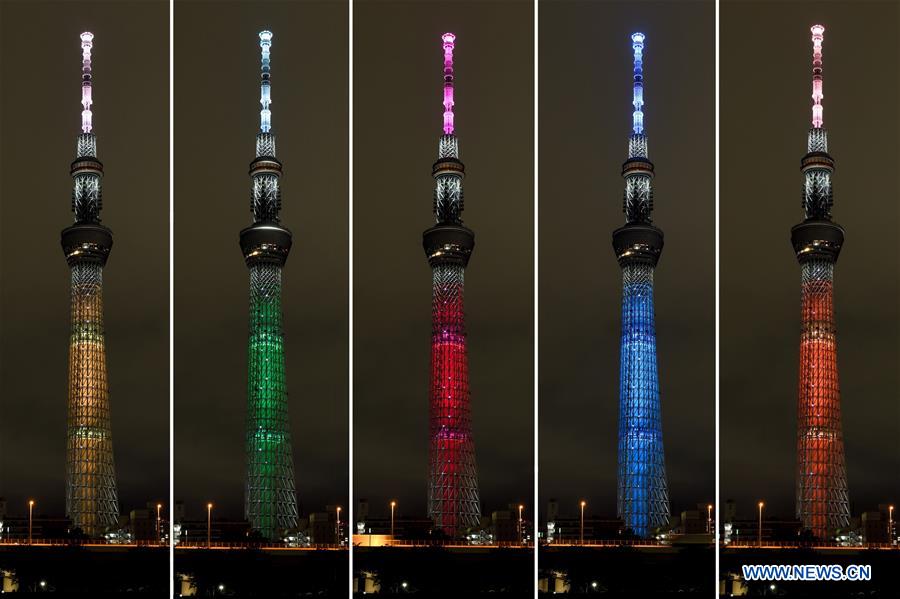The image is a square collage composed of five vertically rectangular, full-color photos of the same building, arranged side by side with a vertical white line dividing each photograph. Taken outdoors at night using artificial lighting, the building is a tall, slender, glass-clad tower with a pointed top and an observation deck. The colors of the building's lights vary across the five images, showcasing yellow, green, red, blue, and orange from left to right. The dark sky has an olive tint, and at the bottom of each image, streets and streetlights are visible, appearing much smaller in contrast to the towering structure. The website www.news.cn is prominently displayed in the lower right corner. The various lighting on the building creates a striking display against the nighttime backdrop.